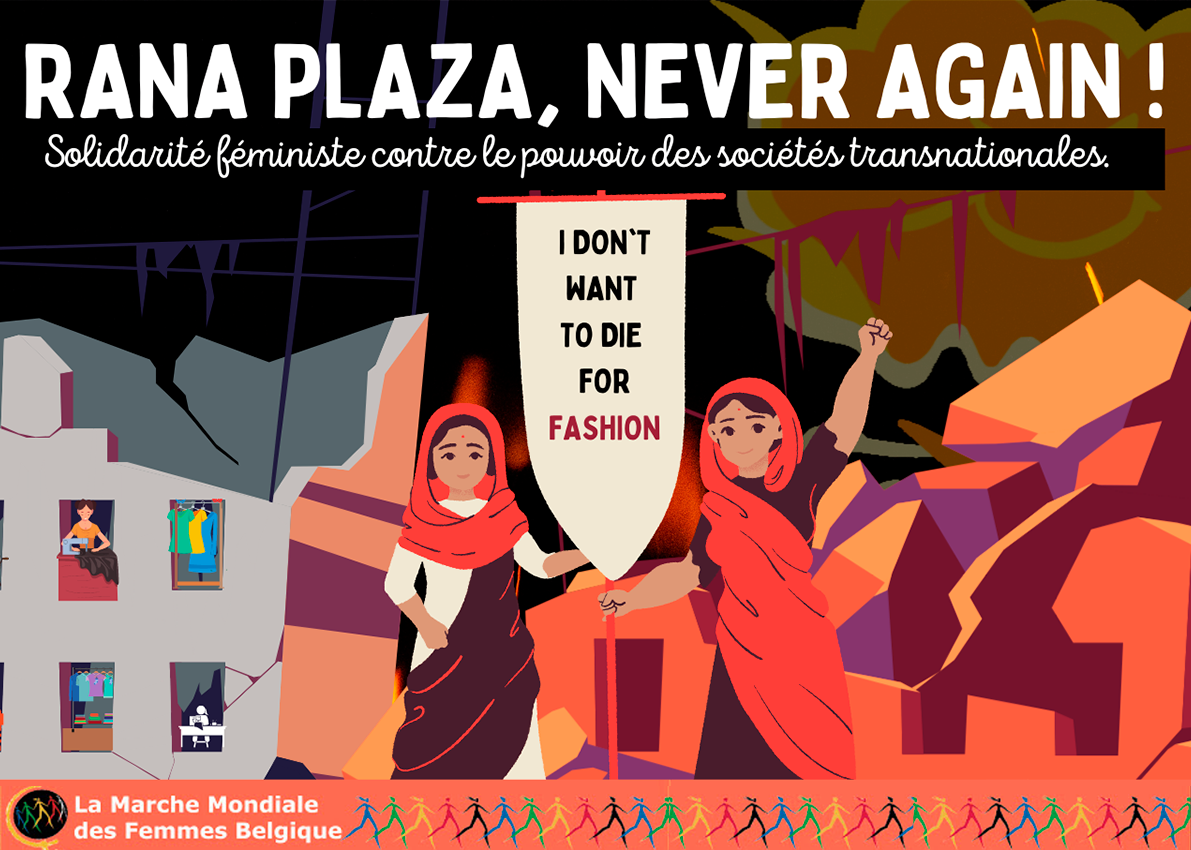This vibrant cartoon-style image is a protest poster depicting a powerful message against the tragic Rana Plaza disaster. Dominating the top of the image, bold white text proclaims, “Rana Plaza, never again!” just above another line of text in French that reads, “Solidarité Féministe Contre Le Pouvoir des Sociétés Transnationales.” At the heart of the image, two women dressed in traditional Bangladeshi attire with red headscarves hold a banner shaped like a flag, with a stark statement in black and red text, “I don't want to die for fashion.”

The woman on the left stands defiantly; meanwhile, the woman on the right raises her fist in solidarity. Behind them, the chaos of their surroundings is dramatically illustrated with broken, crumbling buildings, one still bearing windows and hanging garments. The vibrant hues of orange, purple, and red that color the background contrast sharply with the dark black patches possibly representing dripping blood or shadows of despair.

At the bottom of the image, an orange banner features multicolored stick figures running together, symbolizing unity. This motif is echoed in a black circular logo on the bottom left. Supporting text in French, including “La Marche Mondiale des Femmes Belgiques,” further punctuates the image, linking it to global feminist and labor solidarity movements. The overall poster conveys a poignant and urgent call for change, echoing the voices of women who refuse to give their lives for the fashion industry.